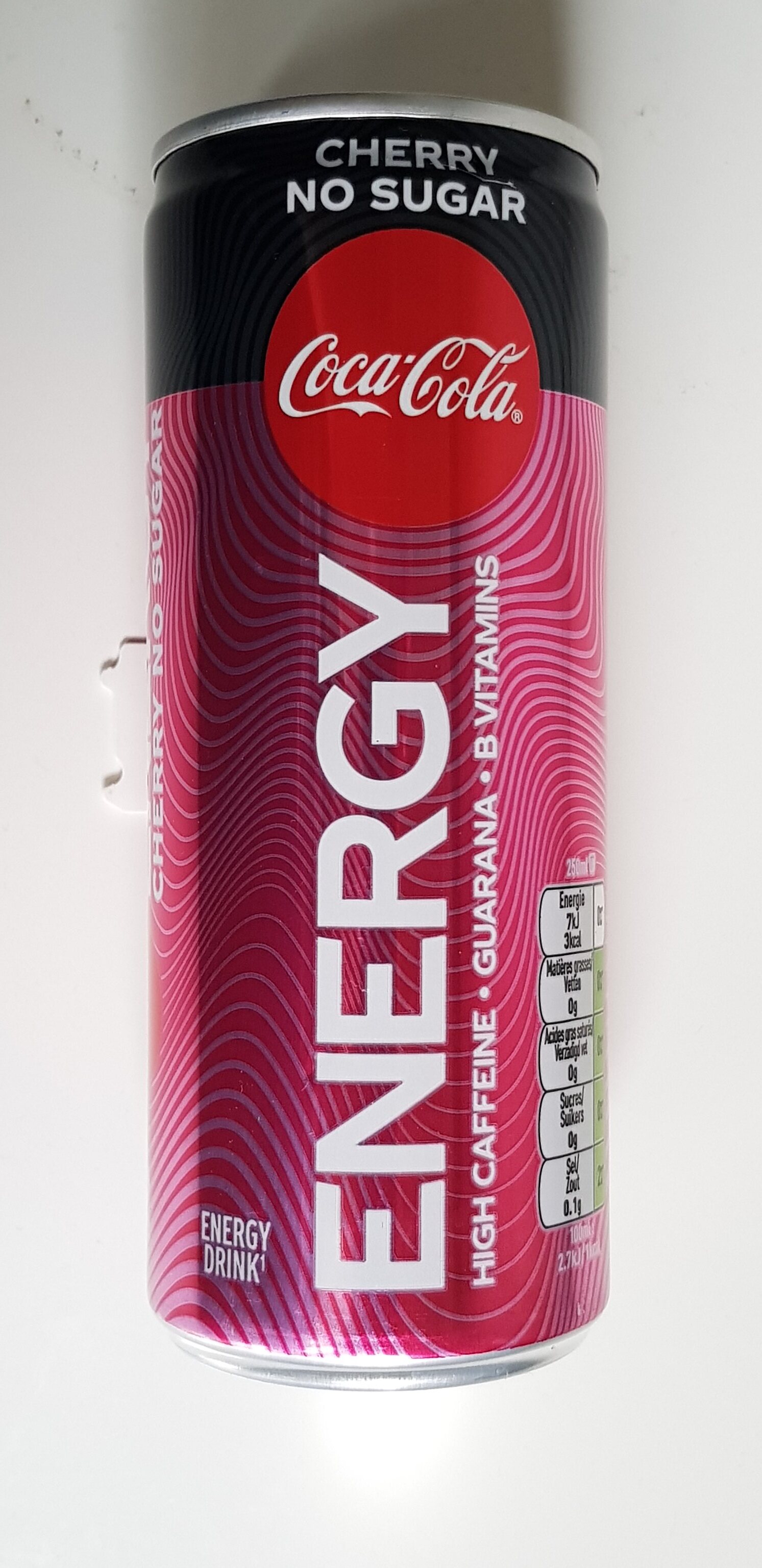This is a close-up image of a Coca-Cola Cherry No Sugar Energy Drink can, lying on its side against an all-white background. The can has a striking design, with the top 20% of it being black, which features the text "Cherry, No Sugar" in white letters. Below this section, the iconic Coca-Cola logo is presented in white cursive within a red circle. The remaining 80% of the can is a vibrant maroon-red color adorned with intricate wavy lines that span the length of the can, creating a ripple effect. Prominently displayed in bold white text along the length of the can is the word "Energy." Beneath this, smaller white text lists the key ingredients: "High Caffeine," "Guarana," and "B Vitamins." The bottom part of the can mentions "Energy Drink" in white. Small white squares indicating nutritional information are visible but unreadable in the image. The overall composition reflects a sleek and modern design intended to catch the consumer's eye.